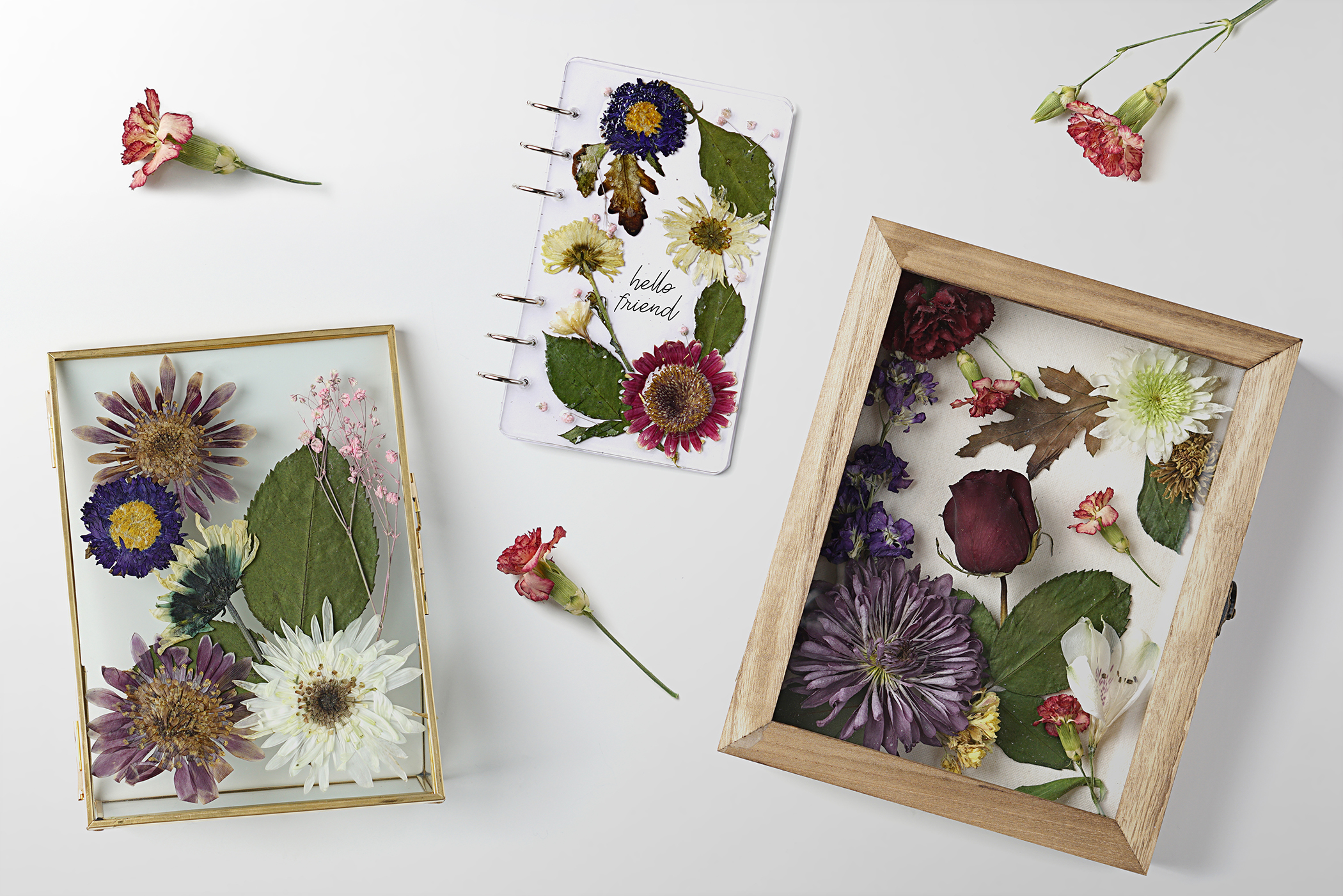The photograph showcases an arrangement of floral art on a white background, comprising three main elements. On the left side, a fine-framed picture displays an assortment of dried flowers and leaves, featuring a prominently large purple flower, delicate white blooms, and earthy green foliage. Centrally positioned is a white, spiral-bound notebook with the greeting "Hello Friend" on its cover, adorned with an array of blue, white, and red flowers. To the right, a wooden-framed picture includes a combination of purple flowers, a central rose, and several green leaves, providing a harmonious contrast. Scattered throughout this layout are three individual red flower sprigs, enhancing the overall aesthetic. The intricate details and careful arrangement highlight the beauty of dried botanicals within artful compositions.